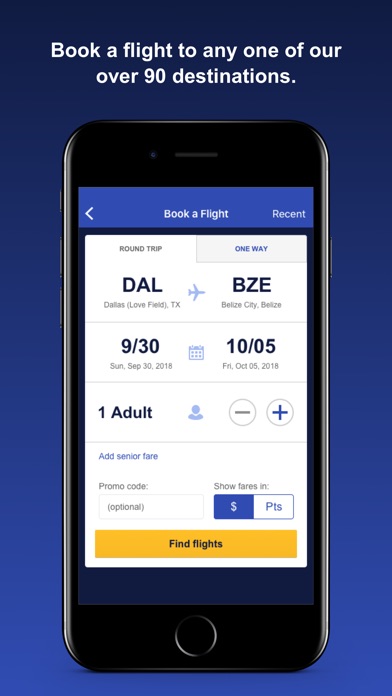The promotional image is designed in a tall, rectangular aspect ratio with a vibrant blue background. It prominently features an older model iPhone standing upright, displaying a flight booking app on its screen. Above the iPhone, against the blue background, bold white text reads, "Book a flight to any one of our over 90 destinations."

The iPhone screen captures immediate attention with an open app interface geared towards booking plane flights. A blue banner within the app displays the text "book a flight" accompanied by a left-pointing arrow, indicating a navigation option to return to the previous screen. The app interface features a white background, detailing a round trip itinerary: "Dallas, Love Field, Texas (DAL) to Belize City, Belize (BZE)." Beneath this, icons and text specify the travel dates: "Sunday, September 30th, 2018 to Friday, October 5th, 2018" for one adult. The bottom of the iPhone screen features a conspicuous yellow "find flight" button, inviting users to proceed with their booking.